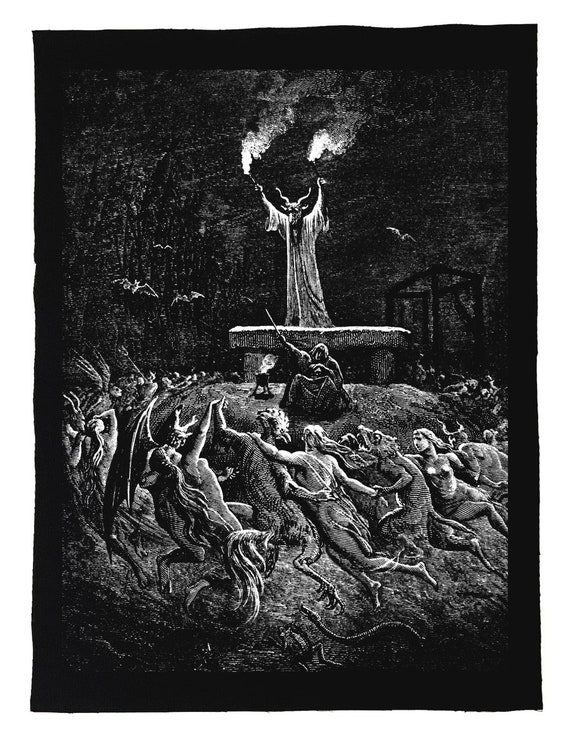The black and white image, resembling an etching or tapestry, is rectangular, with an uneven black border framing it. At the center, a goat-headed devil-like figure, adorned in a white full-body robe, stands on a stone platform resembling a bench with two pillars. Holding smoky torches aloft, the creature's imposing form is accentuated by twisty horns. Surrounding this figure, bats flutter in the dark cave-like background. Below, a robed man sits on the platform with one arm raised, holding a sword or wand, beside a small cauldron. Encircling the mound are tormented, nude humans and bizarre humanoid creatures with unnatural features—some with wings, thin legs, or animal heads like those of iguanas, dogs, or birds. The scene is chaotic and haunting, with serpents on the ground and a sense of agonized movement among the figures, who appear locked in a sinister, infernal dance.